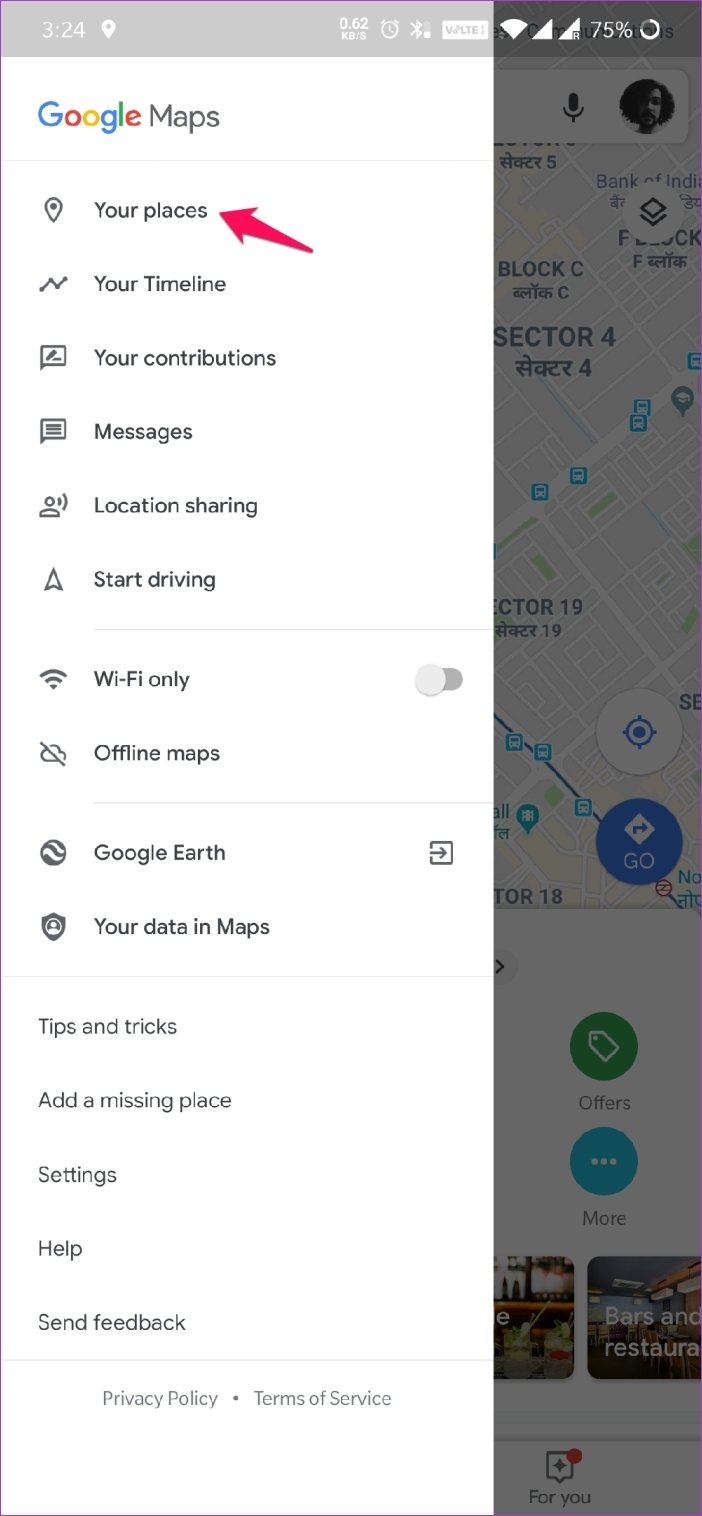The image appears to be a screenshot from a mobile device, such as a phone or tablet, as indicated by the icons and time displayed in the upper left corner, showing 3:24. The status bar includes various icons: a small "Google" logo, a location icon, a download speed indicator, a clock, Bluetooth, LTE for cellular service, Wi-Fi, and a battery at 75%.

Dominating the screen is an overlay from Google Maps, which occupies the majority of the display. This overlay lists several options: "Your places," "Your timeline," "Your contributions," "Messages," "Location sharing," "Start driving," "Wi-Fi only," "Offline maps," "Google Earth," "Your data in Maps," followed by "Tips and tricks," "Add a missing place," "Settings," "Help," "Send feedback," "Privacy Policy," and "Terms and conditions." 

In the background, partially obscured by this menu, is the Google Maps interface itself. The visible portion of the map shows labels such as "Sector 4," "Block C," and "Sector 19," interspersed with Asian characters, likely Japanese. There are also faint, partially visible buttons labeled "Offers" and "More."

The screenshot’s context and content suggest that the user has opened the Google Maps app and accessed the menu, which is now displayed over the map of an Asian locale, potentially in Japan, as inferred from the lettering.